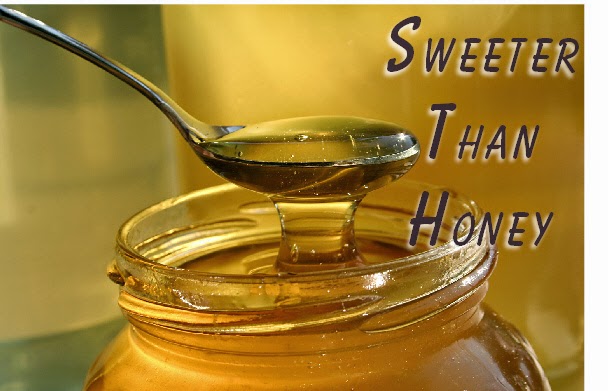The photograph showcases a close-up of a jar of honey with its lid removed, revealing a spoonful of rich, amber-colored honey being drawn out. The silver spoon is positioned towards the top left, overflowing with viscous honey that trails back into the wide-mouthed, clear screw-top jar below. The background features a blend of golden honey hues and light sage green, creating an artistic and slightly blurred effect that accentuates the subject. To the right, in large, dark gray hand-markered font with a light white shadow, is the phrase "sweeter than honey." The lighting in the image is optimal, highlighting the golden tones of the honey and adding to the overall high quality of the photograph, though the text's quality appears somewhat lower by comparison.